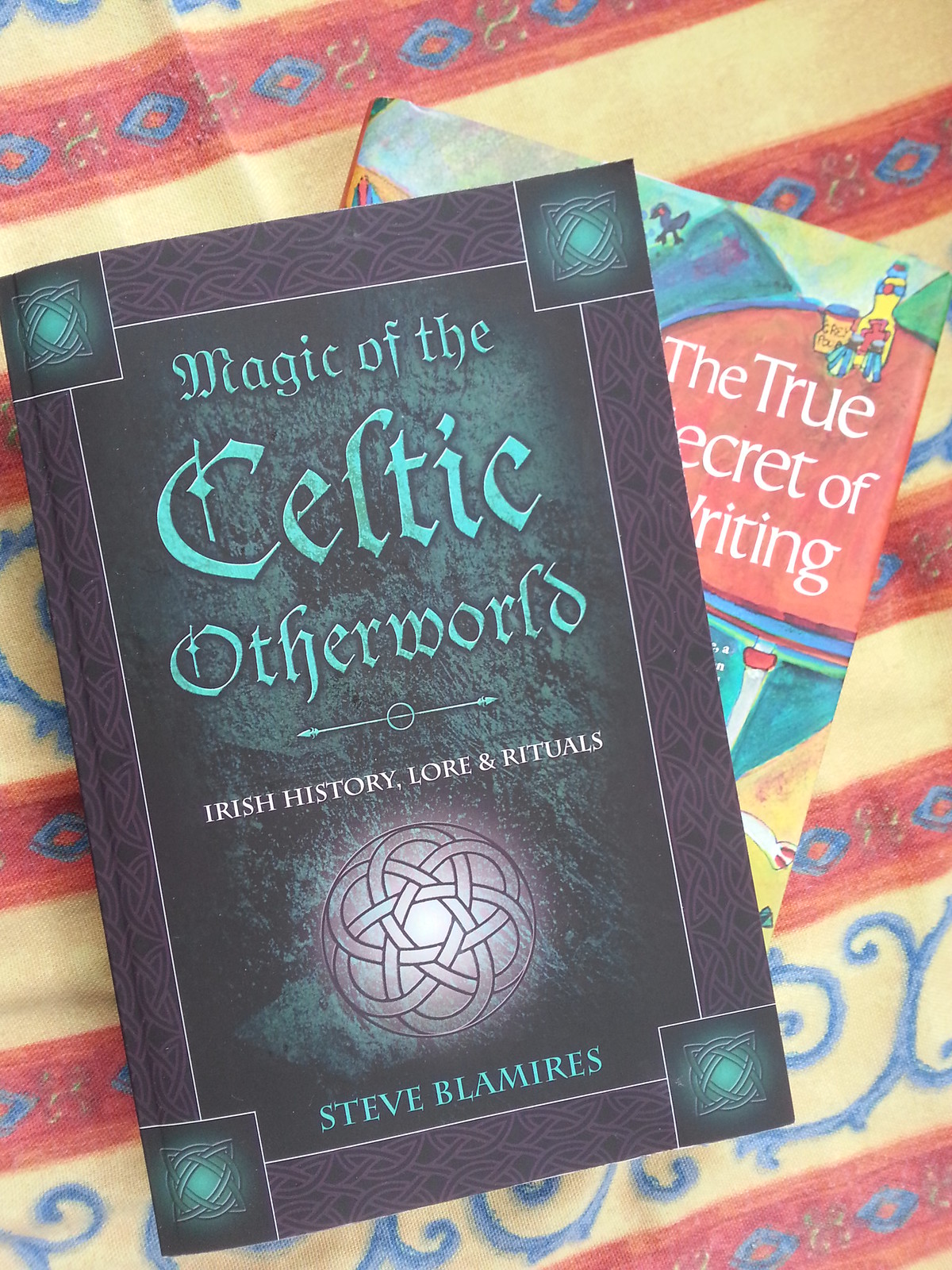The photograph shows an overhead view of two books placed on a colorful tablecloth adorned with a cream base and blue diamond patterns interspersed with red and yellow designs. The book in the foreground prominently features the title "Magic of the Celtic Otherworld" in a striking green font set against a black and dark green background. Below the main title, a smaller white silver font states "Irish History, Lore, and Rituals". A distinctive Celtic logo resembling crisscrossing ovals or a ball of yarn is centrally placed with a subtle glow, and beneath this, the author's name "Steve Blamires" is written in light green text. Each corner of the foreground book is adorned with squared Celtic knot designs. Partially visible beneath the Celtic-themed book is a second book titled "The True Secret of Writing". This underlying book displays a colorful palette, likely portraying a design akin to a crayon or a child's drawing, though much of it is obscured. The overall setting on the patterned tablecloth enhances the scene’s vibrant and textured appearance.